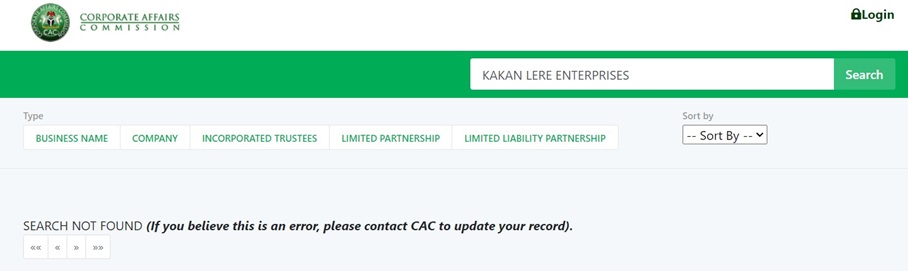At the top of the image, the text reads, "Corporate Affairs Commission," with "Corporate Affairs" underlined and "Commission" spaced out, stretching the letters apart. To the left of these words is the emblem for the Corporate Affairs Commission (CAC). The logo is blurred but appears as a green circle with a gold dish inside. It seems to depict a torso adorned with a necklace and flanked by white snakes on both sides.

On the far right side, there's a login section featuring a small lock icon below it. Below the emblem, there is a green bar with a search box. The text in the search box reads, "CAC and Larry Enterprises" and "KKN LERE" underneath in a lighter gray box. This box contains the placeholder text "Type," and below it are buttons labeled with "connect."

The interface includes options such as "Business Name" in green, "Company Incorporated," "Trustees," "Limited Partnership," and "Limited Liability Partnership." To the right, there’s a "Sort By" dropdown menu. Below that, there's text saying "search found" in all caps. Italicized and bold text to the right reads, "If you believe this an error, please contact the CAC to update your record."

At the bottom section of the visible part of the website, there are navigation arrows for pagination: a double left arrow, a single left arrow, a single right arrow, and a double right arrow. The rest of the webpage is not displayed and appears blank.